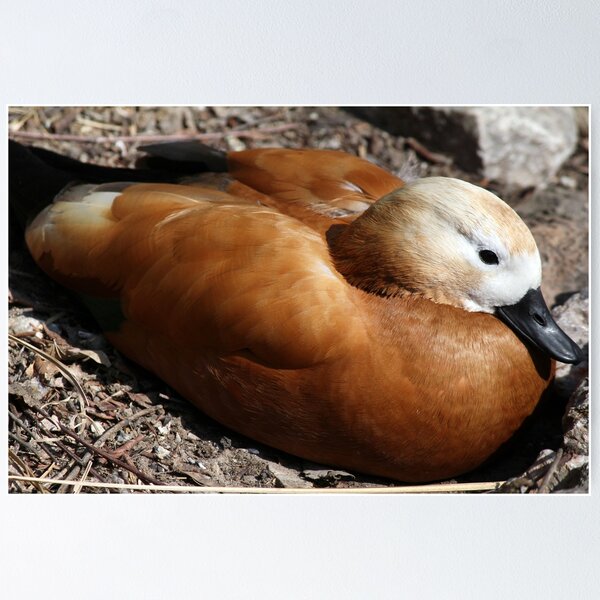A daytime outdoor photograph with a square format enclosed by a blue border that is thicker at the top and thinner along the sides. The image depicts a duck centrally positioned and lying on a ground covered with dead vegetation such as twigs, bare dirt, and small pebbles. The duck has a white head with tan hues, a prominent black bill, and black eyes. Its body is predominantly covered in soft brown feathers, with the tail feathers displaying a touch of cream white that fades into the brown. The bird appears to be resting with its head tucked in, suggesting it might be cold. To the upper right and lower right of the image, there are gray rocks, adding natural elements to the otherwise bare foreground.